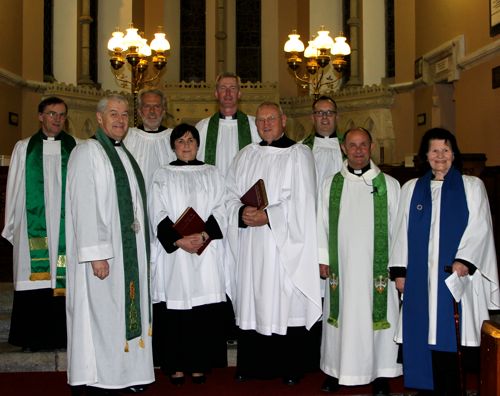In this indoor photograph taken inside a church, nine individuals are standing closely together, all dressed in white religious robes, likely members of a church choir. Some wear traditional priest's collars, while others have shiny satin stoles in various colors draped over their shoulders—most in green and one woman notably in blue. Two individuals in the center hold dark books with their hands clasped in front of them. The backdrop features ornate walls striped in gray, black, tan, and gold, coupled with elegant designs. Above them, on either side, are wall-mounted light fixtures reminiscent of chandeliers, each fitted with multiple bulbs. A rich red rug lies underfoot, adding to the solemn and formal ambiance of the scene.